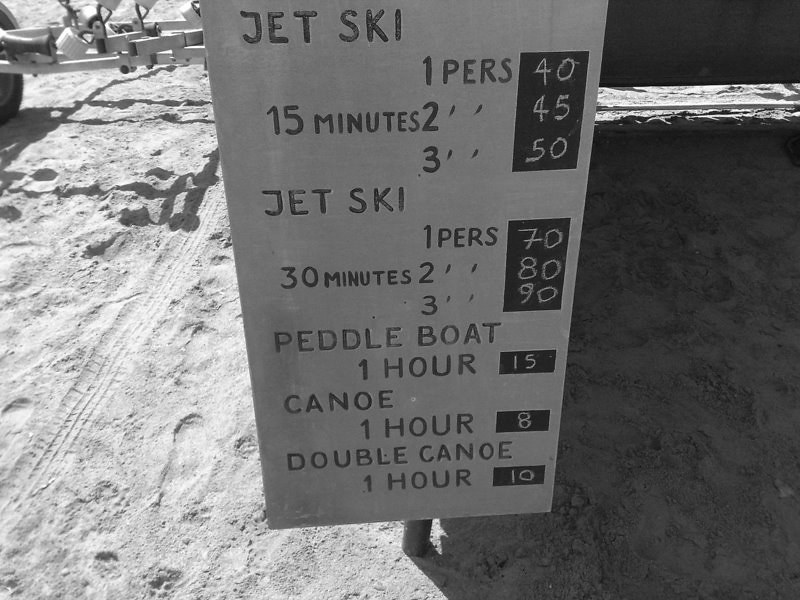The image depicts a black-and-white photograph, capturing a serene outdoor setting with a light snow cover blanketing the ground and visible footprints imprinting the surface. Centrally located within the slightly downward-angled landscape-oriented shot, a white sign with black lettering stands mounted on a vertical post. The left side of the scene remains well-lit, while the right side fades into shadow.

The prominently featured sign displays various rental rates and time increments for water activities, specifically jet skiing, pedal boating, and canoeing. At the top of the sign, it states "Jet Ski, 1 PERS." Below, in a chalkboard section, it lists the prices: 
- 15 minutes: $40 for 1 person, $45 for 2, and $50 for 3 people.
- 30 minutes: $70 for 1 person, $80 for 2 people, and $90 for 3 people.

Further details at the bottom of the sign indicate additional rental rates for other activities:
- Pedal boat: 1 hour for $15.
- Canoe: 1 hour for $8.
- Double canoe: 1 hour for $10.

The presence of a trailer hitch in the background hints at the functional aspect of this recreational spot, situated amidst a tranquil, snowy environment, evoking a sense of nostalgic simplicity through its representational realism style.